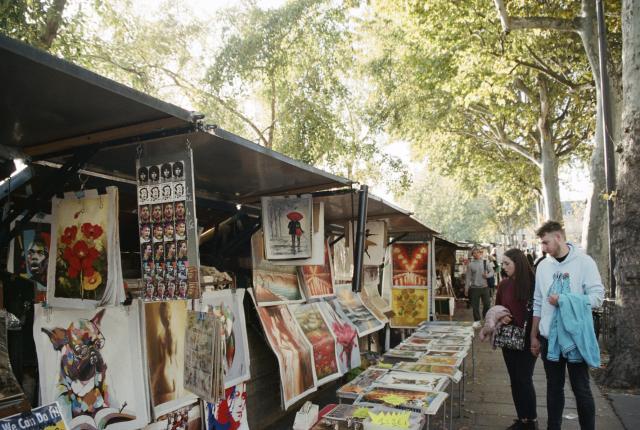This detailed image captures a bustling street fair on a sunny city sidewalk amidst a canopy of lush, green trees in full bloom, suggesting a spring or summer setting. Numerous vendors line the street, displaying a diverse array of colorful prints and paintings, including depictions of flowers, a dog, a nude woman, various faces, famous people, abstract art, and scenic outdoor landscapes. Towards the bottom left, the prints are more distinguishable, while they blur into an assortment further down the street. Dominating the foreground on the right side, a couple is scrutinizing the artwork: the man is in a white hoodie holding a light blue jean jacket, with black jeans; next to him, the woman, with long straight brown hair, wears a burgundy sweater, black pants, black shoes, and carries a crossbody purse with a brown sweater draped over her arm. Both are engrossed in the art, their heads bowed in contemplation. In the background, other visitors and vendors add to the vibrancy of the scene, with sunlight filtering through the verdant trees, providing a picturesque and lively atmosphere.